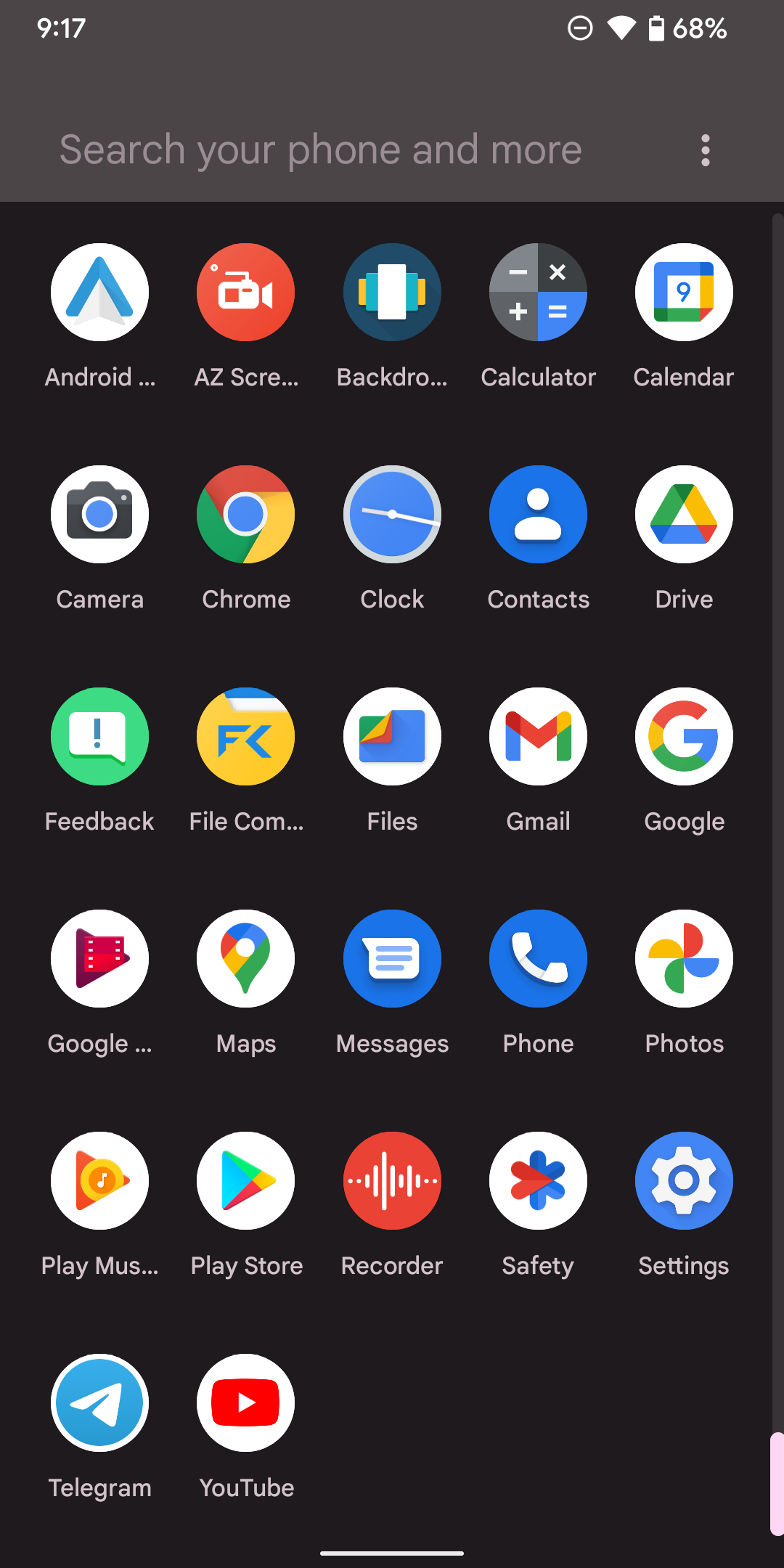The image depicts a smartphone with a prominent gray strip at the top of the screen. In the upper left corner of this strip, the time is displayed as 9:17. The upper right corner features an icon resembling a circle with a line through it, indicating privacy or "Do Not Disturb" mode, alongside Wi-Fi signal bars and a battery percentage of 68%.

Beneath this gray strip, there is a search bar that reads "Search your phone and more," with a vertical three-dot menu icon on the far right. The primary background of the phone's screen is black, providing a stark contrast to the colorful app icons arranged below.

The app icons are organized into a grid, consisting of five icons per row and six rows in total, though the final row contains only two icons. The apps present in each row are as follows:

1. **First row:** Android, AZ Screen Recorder, Backdrop, Calculator, Calendar
2. **Second row:** Camera, Chrome, Clock, Contacts, Drive
3. **Third row:** Feedback, File Commander, Files, Gmail, Google
4. **Fourth row:** Google Maps, Messages, Phone, Photos
5. **Fifth row:** Music, Play Music, Play Store, Recorder, Safety, Settings
6. **Sixth row:** Telegram, YouTube

At the very bottom of the screen, there is a white line centered horizontally, which appears to function as a gesture navigation indicator. Positioned towards the bottom right is a light pink bar, suggesting that the user has scrolled to the bottom of their app list.